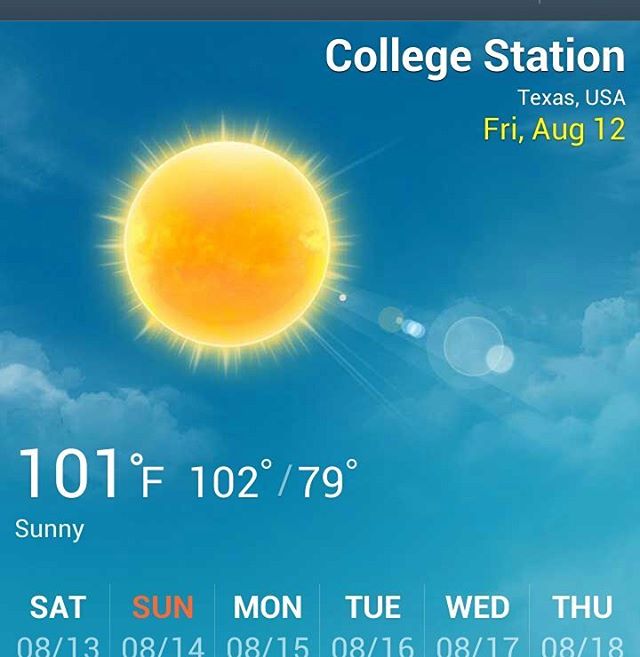This rectangular screenshot, likely taken from an Android mobile device, serves as a detailed weather forecast. The image features a subtle dark navy blue or gray header at the top. Below this header, the background transitions into a vivid depiction of a blue sky scattered with light white clouds, starting approximately mid-image. Dominating the upper left portion of the image is a large bright yellow sun radiating sunbeams. 

In the upper right corner, bold white text reads "College Station," with "Texas, USA" just beneath it in a smaller font. Directly below this, in gold print, it displays "Friday, August 12th." Centrally positioned beneath the sun, the forecast shows "101 degrees Fahrenheit" in large white text, followed by "102 degrees / 79 degrees" and "sunny" in smaller white text.

The lower section of the image lists the upcoming days of the week, from Saturday to Thursday, each aligned horizontally. "Saturday" (08/13) appears in white, while "Sunday" (08/14) stands out in orange. Continuing to the right, "Monday" (08/15), "Tuesday" (08/16), "Wednesday" (08/17), and "Thursday" (08/18) are written in white, each accompanied by their respective dates in light blue print.